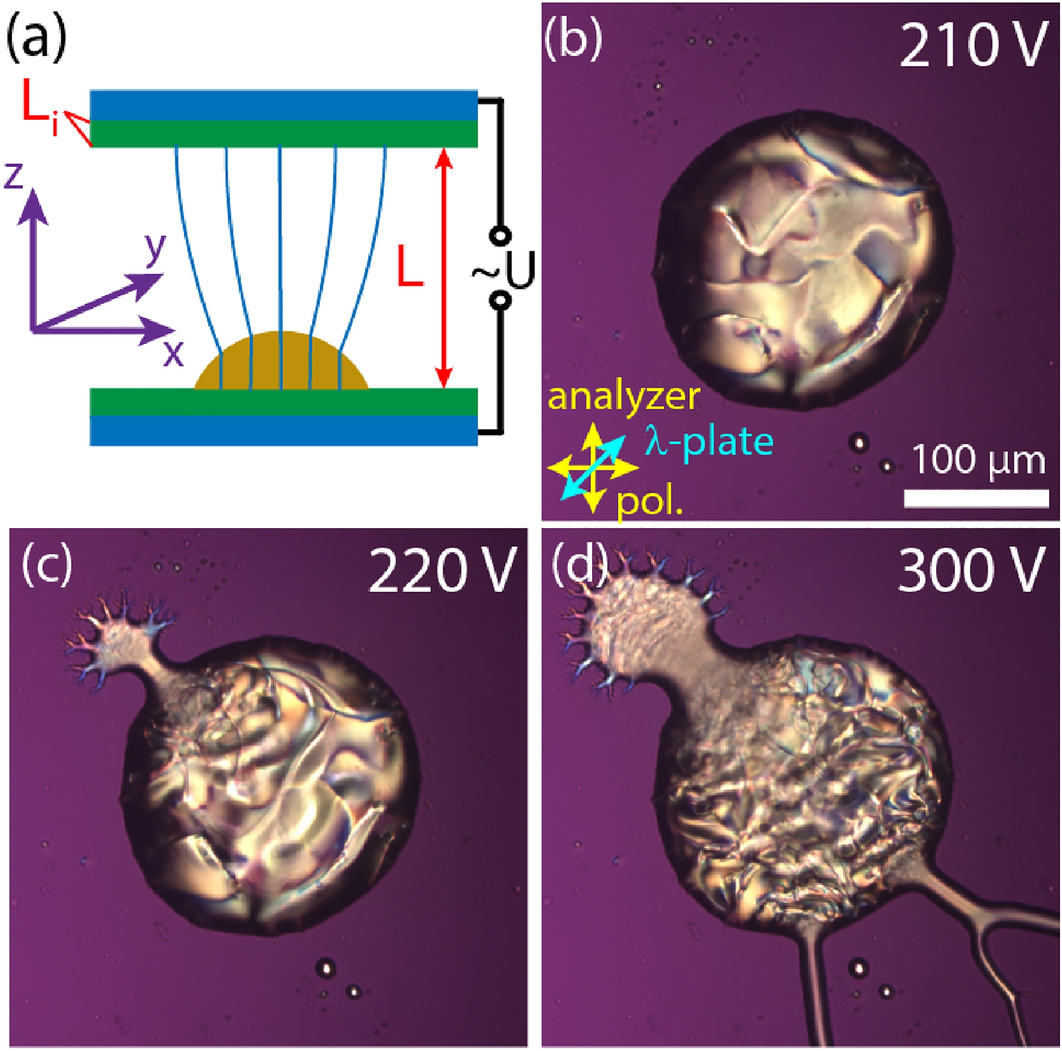The image is divided into four distinct squares, each labeled with a letter (A, B, C, and D) and containing intricate visual and textual details, primarily in purple, blue, green, and red hues. At the top of the image, square A features blue and green horizontal stripes, while the bottom has green and blue vertical stripes. It includes the letter 'L' with a base indicating 'I' and red lines projected sideways, alongside an X, Y, and Z axis shown in purple on the left side. To the right, there's the letter 'U' with the label "About You" and a curly or approximately symbol. A sun illustration in the center emits four vertical, slightly curved lines upward through the green bars.

Square B, positioned on the right, contains the text "210V" and labels such as 'Analyzer,' 'Lambda Plate,' and 'POL' in the lower left corner. It features multi-directional arrows similar to an axis, a scale indicating 100 micrometers, and a texture resembling melted metal, possibly of microscopic origin, possibly a nerve.

Squares C and D, found on the left and right of the picture, display textures similar to square B, resembling melted metal with nerve-like projections. Square C is noted as "220V" and square D as "300V." This detailed image likely serves an educational purpose, potentially illustrating cellular abnormalities or structures under a microscope, and emphasizes the complex visual patterns and measurements involved in microscopic analysis.